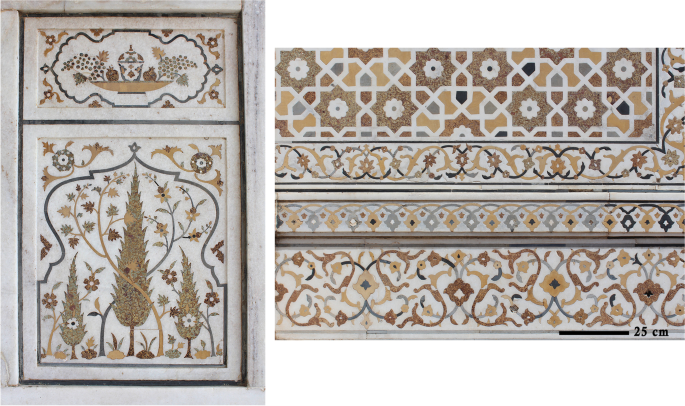The image presents two distinct artistic pieces set against a white background. The left side features a framed art piece with a weathered wood look, enclosing two hand-painted tiles. The larger bottom tile depicts three abstract pine trees, the middle tree being the tallest and flanked by two shorter ones. The scene, rendered in muted tones of green, dark and light blue, and gold, includes branches and flowers crisscrossing symmetrically around the trees, with a faint crown-like outline in a bluish-gray hue. The smaller top tile, occupying about a quarter of the frame, portrays a serving dish adorned with hand-painted grapes and an abstract vase in the center, utilizing a subdued palette of gold, yellow, ochre, and blue shades.

On the right side, we see a close-up of another tile, bordered by white wood, characterized by a patchwork pattern of geometric shapes like pentagons, rectangles, and circles. This tile incorporates colors similar to the left piece, including muted blues, grays, browns, yellows, and ochre. A measuring legend at the bottom reads "25 centimeters," offering a sense of the tile's size. Both pieces share a harmonious color palette and exhibit intricate, hand-painted details, creating a cohesive visual narrative.